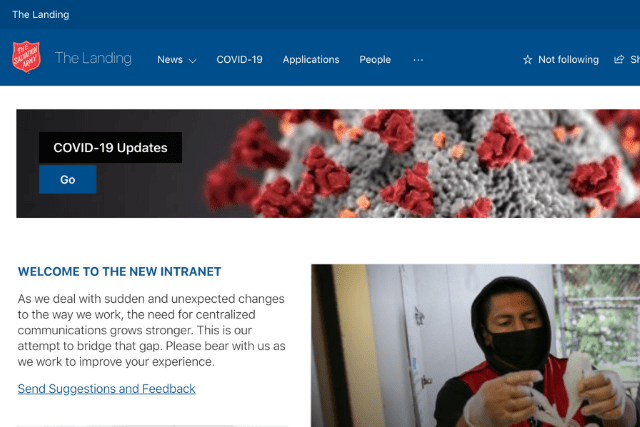This image appears to be a screenshot from a website, likely an internal communication platform or intranet. At the top of the image, there is a blue rectangular banner. In the top-left corner of this banner, the text "The Landing" is prominently displayed in white. Below this, there is a red shield emblem with the words "The Salvation Army" written diagonally in white.

Next to the emblem, the header features additional navigation items. These include:
- "The Landing" in white.
- "News" with a small drop-down arrow.
- "COVID-19" and "Applications."
- "People."

On the far right side of the header, there is a small star emblem followed by the text "Not Following."

Beneath the header banner, there is another rectangle containing the text "COVID-19 Updates" in white, set against a small black rectangular background. Directly below this, a smaller blue rectangle with the word "Go" in white is prominently displayed. 

The central portion of the image includes a graphic of what appears to be a germ or virus under a microscope. The colors in this image are various shades of red, orange, and gray. Below this graphic, there is a welcoming message in blue text: "Welcome to the Intranet."

Followed by the introductory message:
"As we deal with sudden and unexpected changes to the way we work, the need for centralized communication grows stronger. This is our attempt to bridge that gap. Please bear with us as we work to improve your experience." 

Just below this message, there is a blue link that reads "Send your suggestions and feedback." 

To the right of this text, there is a rectangular image of an individual wearing a black mask over their face.